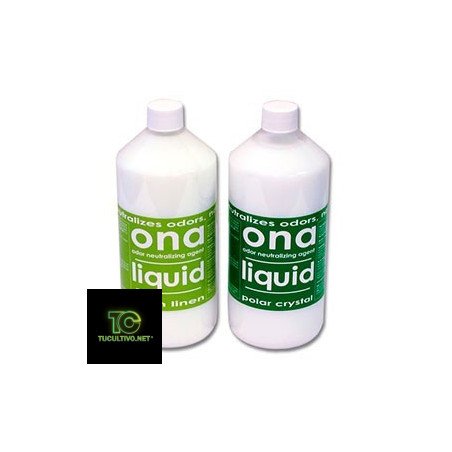The image showcases two white bottles with screw-on caps against a white background. Both bottles are labeled "ONA Liquid," prominently advertising their function as odor neutralizing agents. The bottle on the left features a light green label with the specific scent "Linen," while the one on the right has a dark green label labeled "Polar Crystal." Despite a slight lighting difference making the bottle on the right appear darker, both labels share similar design elements, including a black logo in the bottom left with the text "t-u-c-u-l-t-i-v-o.net."